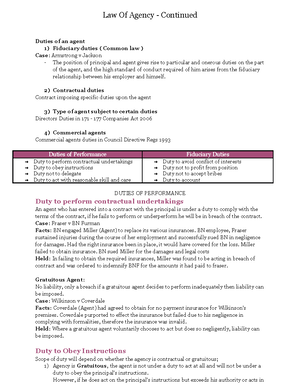**Descriptive Caption:**

The image depicts a screenshot of a document with a formal and detailed layout resembling an academic or professional text. The top of the document features a centered title in black font, which appears to read "Law of Agency - Continued." Immediately below the title, there is a double-spaced gap followed by a bolded line of text, likely serving as a subsection heading, left-indented.

The document continues with a sequence of sections, each introduced by bolded text: the first section starts with a bolded character, possibly "1" or "A," followed by descriptive sentences. This pattern is repeated with subsequent sections, delineated by their bolded headings: a second section, a third composed of two bolded lines, and a fourth similarly styled section, each accompanied by related explanatory text beneath.

In the central part of the document, there is a table spanning two columns. The first row of the table is distinguished by a reddish background with white text, containing four bullet points in each column.

The latter half of the document features text interspersed with bolded words, potentially indicating definitions. It begins with a sentence in a purple or pink font and continues with several paragraphs. The section concludes with additional pink text near the bottom, followed by three to four more lines of standard text.